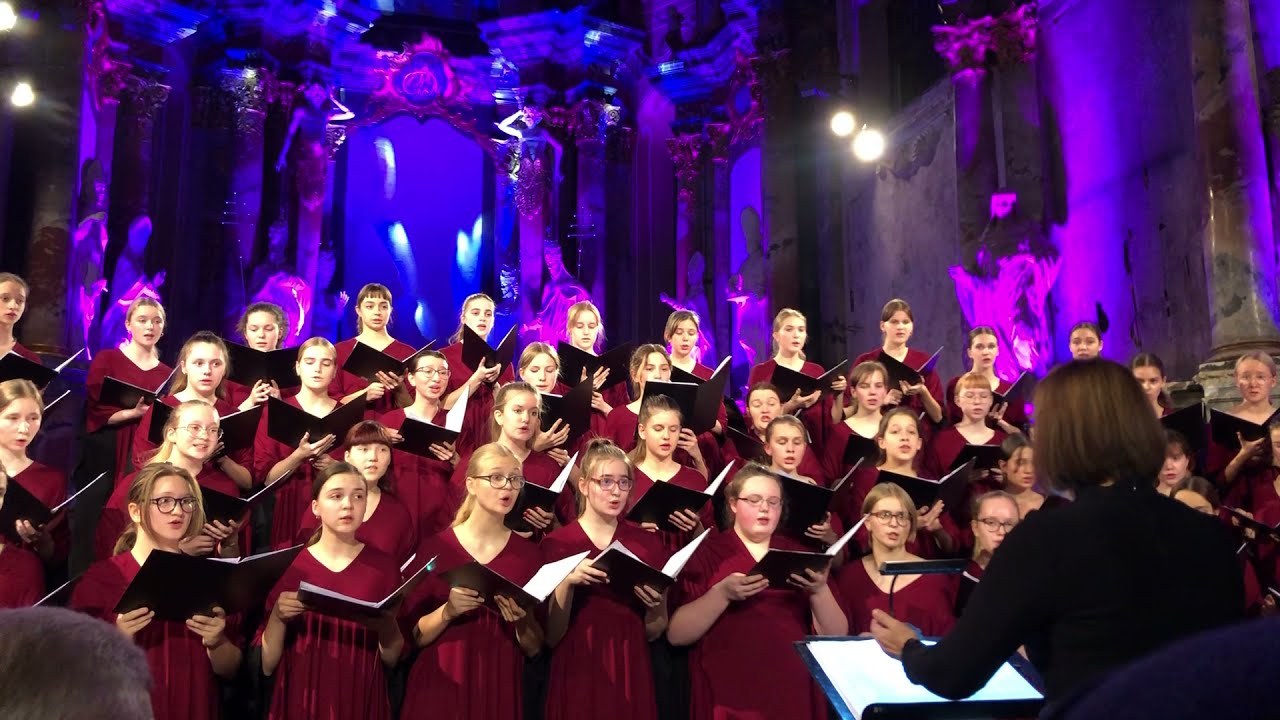The image captures a stunning choir performance set against an illuminated backdrop of decorative columns and statues bathed in pink and blue light. The choir is composed of approximately 40 young girls, all uniformly dressed in elegant red gowns, holding open black music books. The scene is vibrant, with a female conductor positioned at the lower right, facing the choir. She has short dark brown hair styled in a bob cut and wears a black top, guiding the singers with a composed demeanor. Her music score is placed on a stand before her. The setting gives off an event-like atmosphere with intricate details, from the conductor's poised stance to the choir's focused expressions, creating a harmonious blend of music and visual splendor.